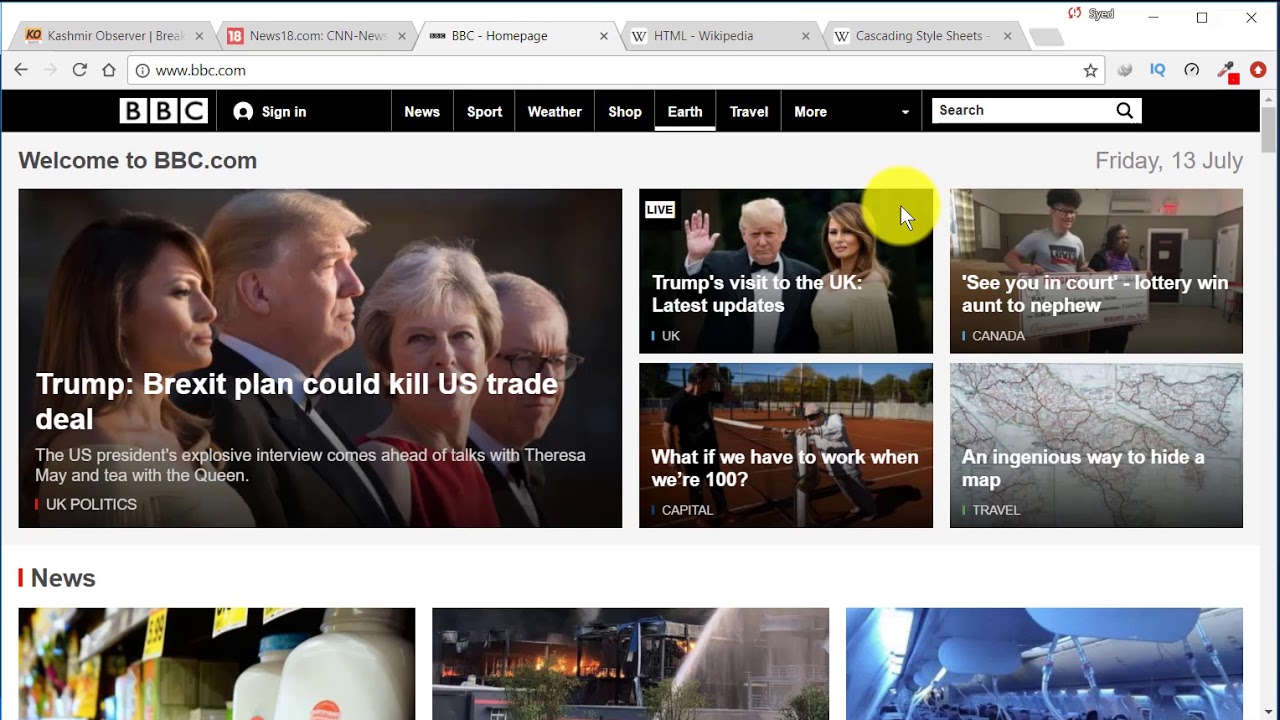The webpage displayed is from BBC's official site, indicated by the URL in the search bar: www.bbc.com. At the top of the browser window, several tabs are open, including Kashmir Observer, news18.com, BBC, homepage, HTML, Wikipedia, and Cascading Style Sheets. The website's header offers navigation options such as sign-in, news, sport, weather, shop, earth, travel, and a dropdown for more content. Additionally, there is an internal search bar available for users to explore BBC's vast array of content.

The main welcome message reads, "Welcome to bbc.com." Below this, a prominent image captures former U.S. President Donald Trump and First Lady Melania Trump, accompanied by two Canadian officials. The headline for this section states, "Re-exit plan could kill US trade deal." 

Adjacent to this is another section highlighting "Trump's visit to the UK," with a picture providing the latest updates on this event. Another intriguing article featuring an elderly worker poses the thought-provoking question, "What if we have to work when we're 100?"

Further down, a section titled "See you in court: Lottery win, aunt to nephew" features an image of two individuals, hinting at a legal dispute over a lottery win between family members. Another small image within the travel section illustrates a unique concept for hiding a map, captioned, "An ingenious way to hide a map."

Underneath the news segment, there are three partially visible images. The first appears to show grocery store shelving with dairy products, likely milk; the second image seems to depict a water geyser in front of a building; and the third image possibly represents the interior of an airplane.